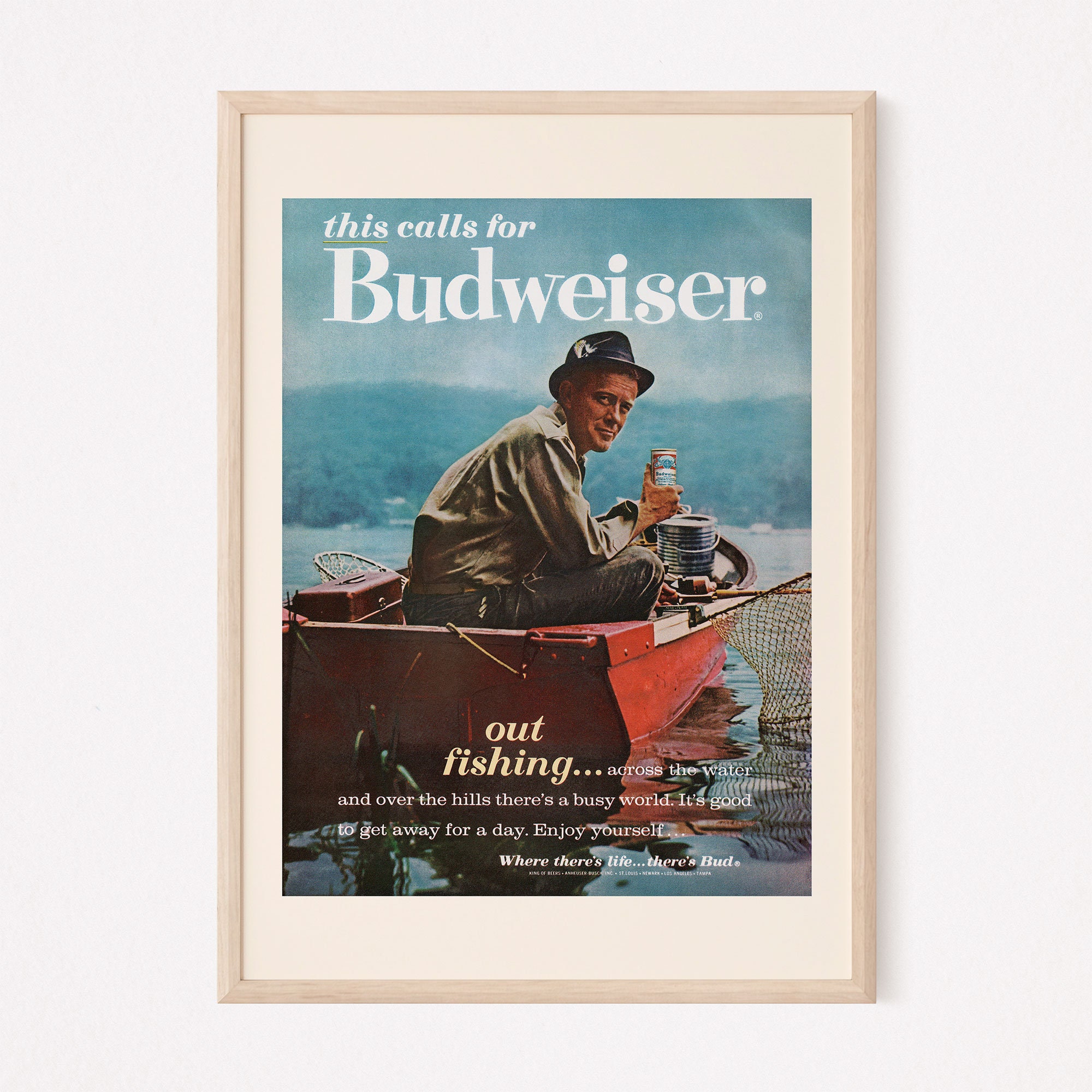This framed advertisement from the 1970s or 1980s features a natural light brown wooden frame with a tan matting, set against a white background. The poster depicts a man sitting in a red boat on a body of water. He is wearing a black hat and a baggy shirt, holding a can of Budweiser beer in his right hand. The background displays a scenic landscape with docks, trees, and foliage. The top of the ad proclaims, "This calls for Budweiser," while the bottom reads, "Out fishing, across the water and over the hills there's a busy world. It's good to get away for a day. Enjoy yourself. Where there's life, there's Bud." Additional fishing gear, including nets and a metal tackle box, are visible in the boat, emphasizing the theme of relaxation and escape from a busy world.